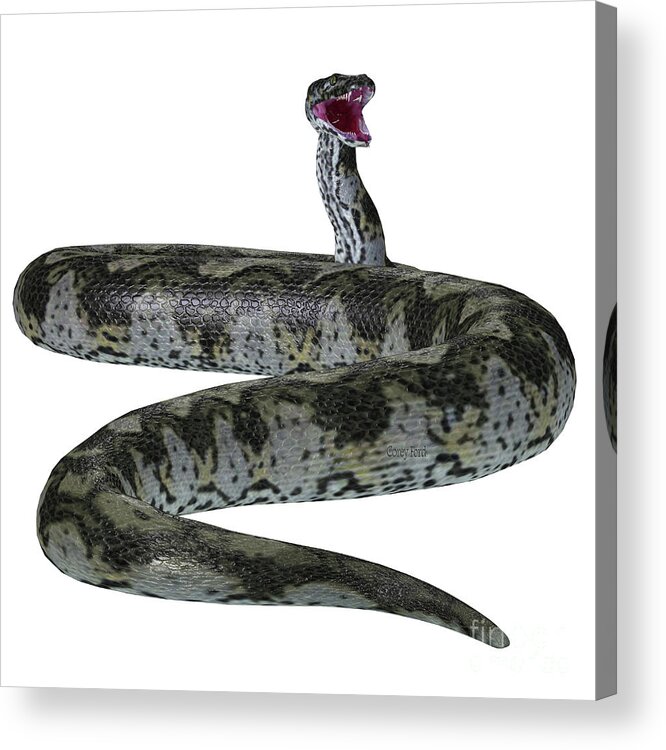The digital artwork displayed on a frayed canvas features a menacing snake poised as if ready to strike, its semi-coiled body highlighting its girthy proportions. The snake's head, unusually thin compared to its thick body, is elevated with its mouth ajar, showcasing a stark red interior that nearly appears purple. Though fangs are hard to discern, the detailed patterning of its dark green, black, and light gray scales, subtly accented with hints of yellow and spots, spans from head to tail. This intricate texture is most vividly illustrated near the head. The snake's body seems to wrap around the right side of the dimensional canvas, offering an added depth to the piece. Against the pure white background, the image takes on a contemporary, almost photographic yet digital quality. At the tail, the word "F-I-N" is legible, accompanied by other smaller, indistinguishable letters near the snake's head, adding an enigmatic textual element to the artwork.